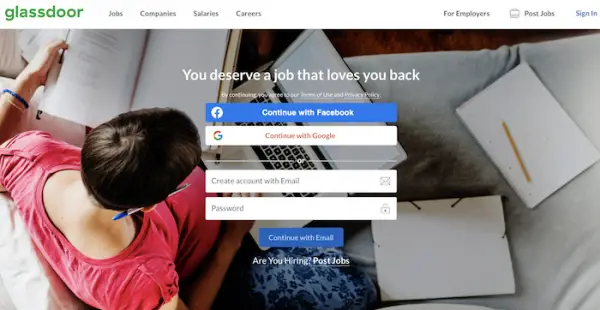This image from Glasdore's emergency website depicts a woman in Bed IV experiencing pain in her right ear. She is multitasking, holding a book in her left hand while using a laptop placed on her lap with her right hand. Several other books are scattered around her on the bed. The website features text that links to various job-related services, such as listing job openings, company information, salary insights, and career resources for employers. The page encourages users with the phrase, "You deserve a job that loves you back," and includes a prompt for users to agree to the terms of use and privacy policy to continue. Options for proceeding include signing in through Facebook, Google, or creating an account with an email and password. There is also a call-to-action for employers, asking, "Are you hiring? Post jobs."